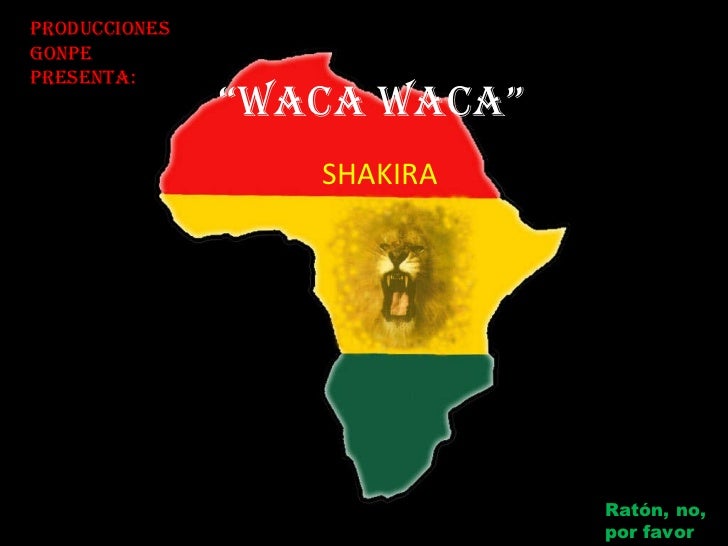The image is a large, rectangular poster with a solid black background. In the upper left-hand corner, there is left-aligned red text that reads "Producciones Gonpi Presenta." The central focus of the image is the outline of the continent of Africa, which is divided into three horizontal sections: red at the top, yellow in the middle, and green at the bottom, all bordered by a white outline. Within the yellow middle section, a roaring lion's head is prominently displayed, with its mouth open wide, showcasing its fangs, tongue, whiskers, and eyes. Across the top part of the continent, within the red section, white capital letters spell out "WAKA WAKA." Directly below in the same red section, yellow capital letters read "SHAKIRA." In the lower right-hand corner of the image, green left-aligned text reads "Raton, no, por favor." The overall design has a bold, graphic style, emphasizing vivid color contrasts and clear text.